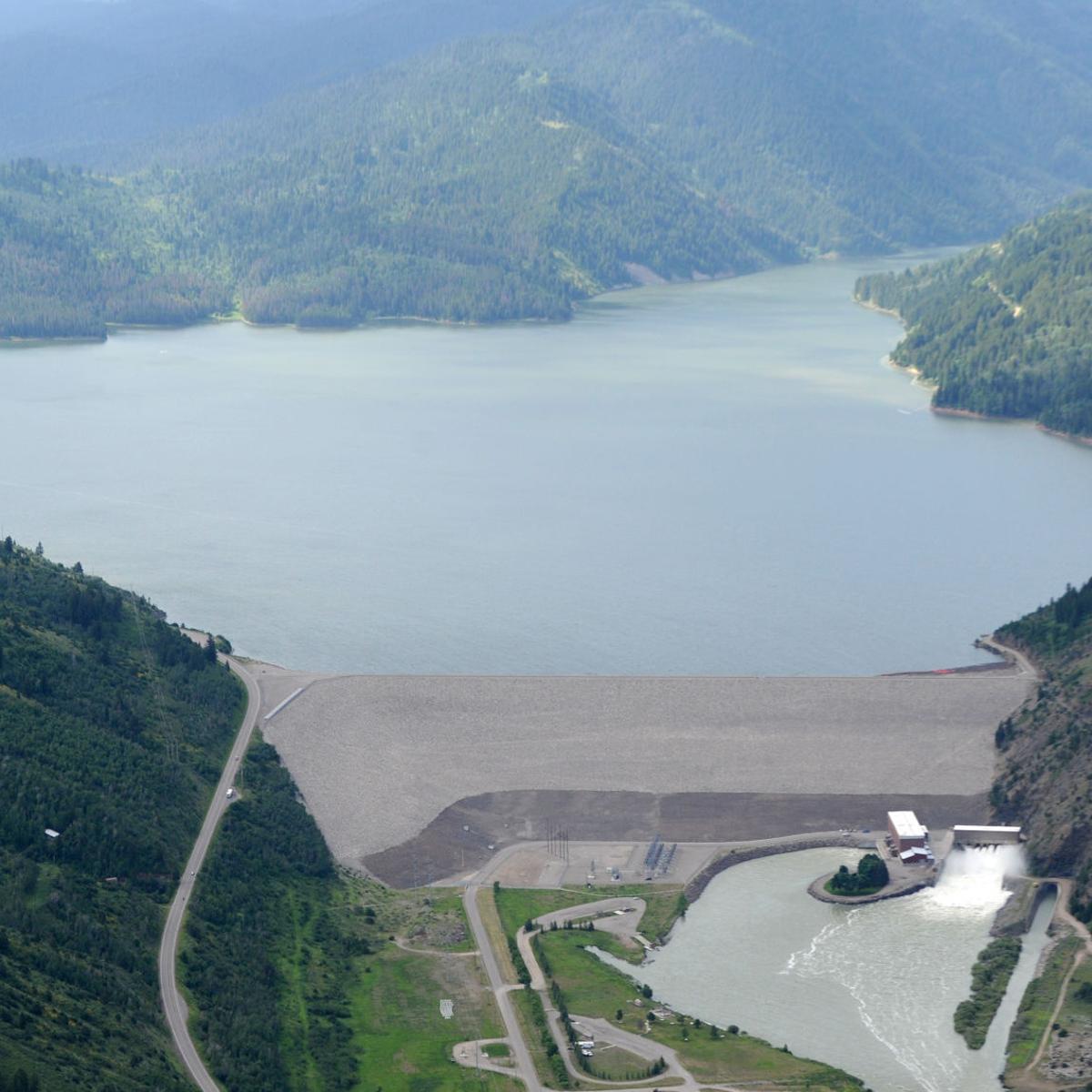In this high-elevation photograph captured under bright sunlight, the central feature is a vast blue reservoir, suggesting it's a man-made lake, with a river visible flowing through the middle to the right. The image is framed by lush green mountains and dense trees that span across the upper background. 

To the left side of the photo, there's a dark green, sloping hill intersected by a winding road, adding a dynamic diagonal element to the landscape. Below the hill, towards the lower third of the image, a cement structure extends into a smaller portion of the lake, functioning as a spillway or dam, which is surrounded by additional blue waters of the lake. A gray boat-like structure sits at the bottom left.

The lower third of the image is dominated by a brownish path, resembling a runway or road with adjacent grassy patches, and it flanked by green spaces and trees. Several roads diverge from this path, particularly leading from the center left to the bottom left, enhancing the intricate network within the landscape. The interplay of different elements creates a richly varied and meticulously detailed outdoor scene.